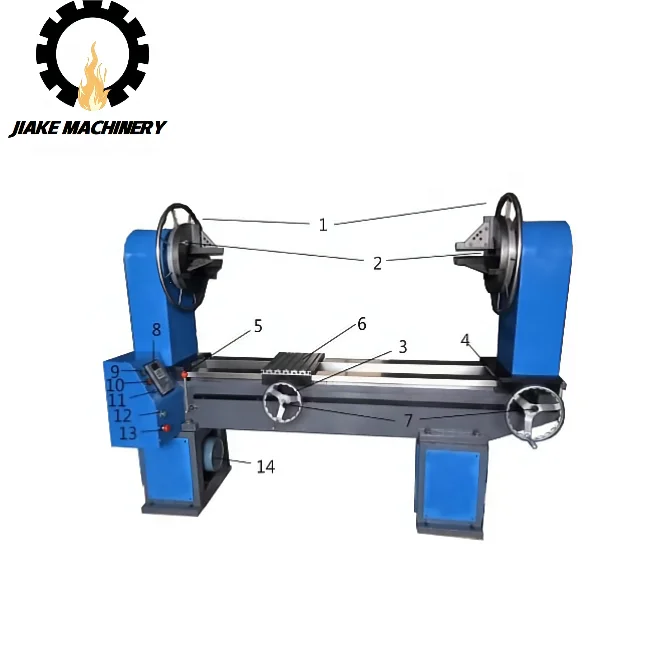This image depicts a piece of manufacturing machinery, prominently featuring a logo in the top left corner. The logo consists of a black cog with a flame at the bottom, colored orange with a yellow center. Below the logo, the black text reads "JIAKE Machinery," spelled J-I-A-K-E. The machinery itself has a predominantly blue and black color scheme with silver and red accents in certain areas. It has a symmetrical design with two arched metal panels on either end, each housing a black wheel flanked by flat pieces. The legs of the machine are black with blue rectangular accents, and the wheels are noted as numbers 1 and 2, respectively. 

The image contains several numbers, up to 14, with lines pointing to various parts, though the parts are not labeled. There are two significant wheels: one on the right side, intended for manual operation, and a smaller, centered wheel attached to a black sliding piece. Additional features include various screws, pulleys, and knobs, adding to the intricate design of the machine. A smaller wheel or button can be observed on the underside of one of the legs, further emphasizing the complexity and multi-functional nature of the device.